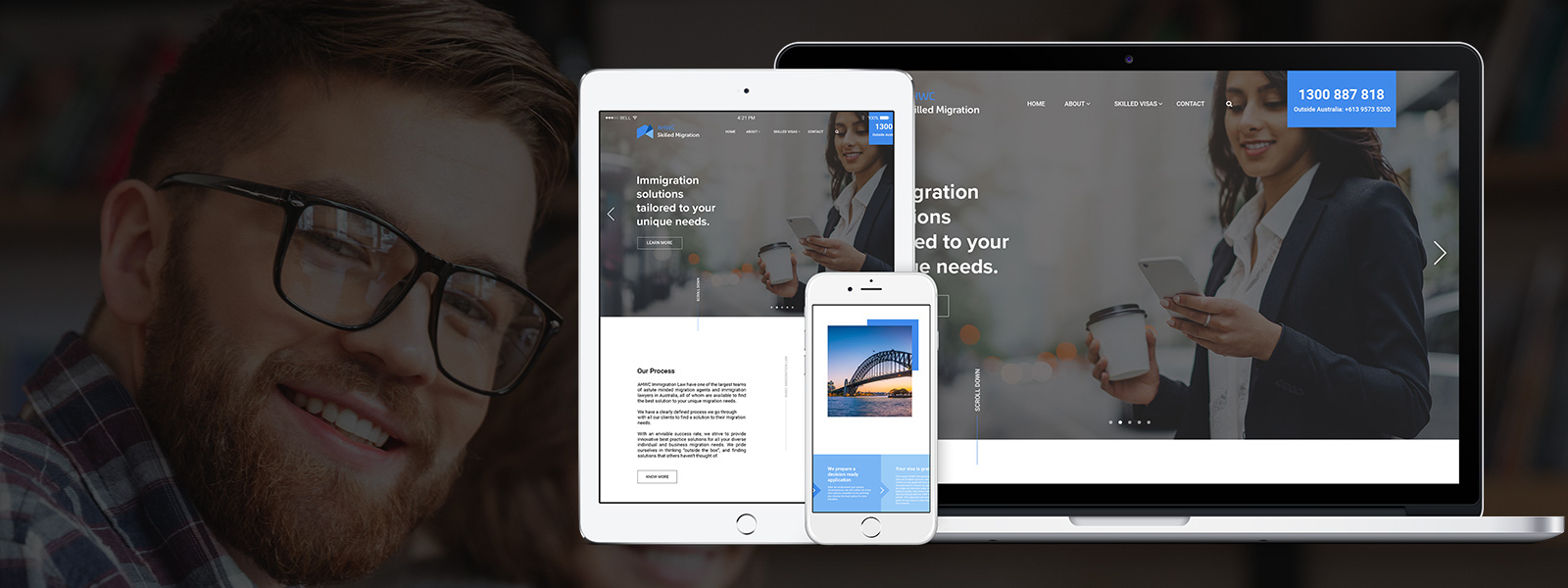A digital image showcases a close-up of a man with glasses and brown hair, wearing a plaid shirt. His head is turned to the side. The image is notably wider than it is tall, emphasizing its horizontal orientation. Beside him, on the same screen, appears a woman dressed in a gray blazer over a white button-down shirt. She holds a phone in her left hand and a coffee cup in her right, her gaze directed downward.

The screen is cluttered with several pop-ups. A prominent blue pop-up displays a phone number at the top. Below it, there is an image of a white iPad displaying the same ad. Within this ad, there's a picture of a bridge with a blue box containing a description underneath. Additionally, a white iPhone is superimposed on top of the iPad image, showing the same bridge picture and description. The overall scene is congested with visual information, highlighting the multiple layers of digital advertisements.